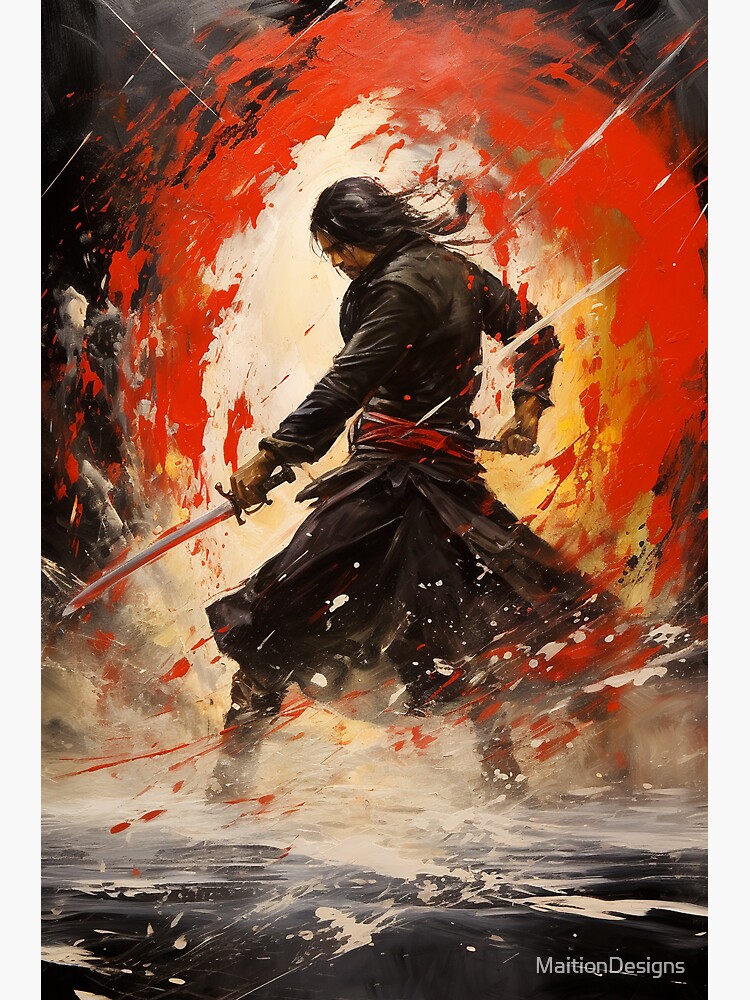This meticulously detailed painting, labeled "Mation Design" in the bottom right corner, showcases a dramatic action scene featuring a dynamic swordsman reminiscent of a Spanish samurai. The subject, who stands with his back facing the viewer and his face slightly turned to the left, wields a blade in his left hand and reaches for another sword holstered behind his back with his right. He sports a long, dark, almost skirt-like jacket, accessorized by a red tie-like belt around his waist. His dark hair, tied into a braid, complements his brown skin complexion.

The artwork’s background is a striking contrast of colors: a predominantly black backdrop encircling a vivid orange, with a white center that highlights the swordsman. This swirling color motif extends into splashes of white and reddish-orange paint, creating a whirlwind effect around him. The ground beneath his feet appears damp, indicative of either water or the aftermath of a battle, highlighted by a circular spray of blood around the blade in his left hand. This masterful blend of movement and color, with intentional splatter patterns, conveys a sense of powerful motion as if the act of unsheathing his sword itself orchestrates the chaos of colors and elements surrounding him.